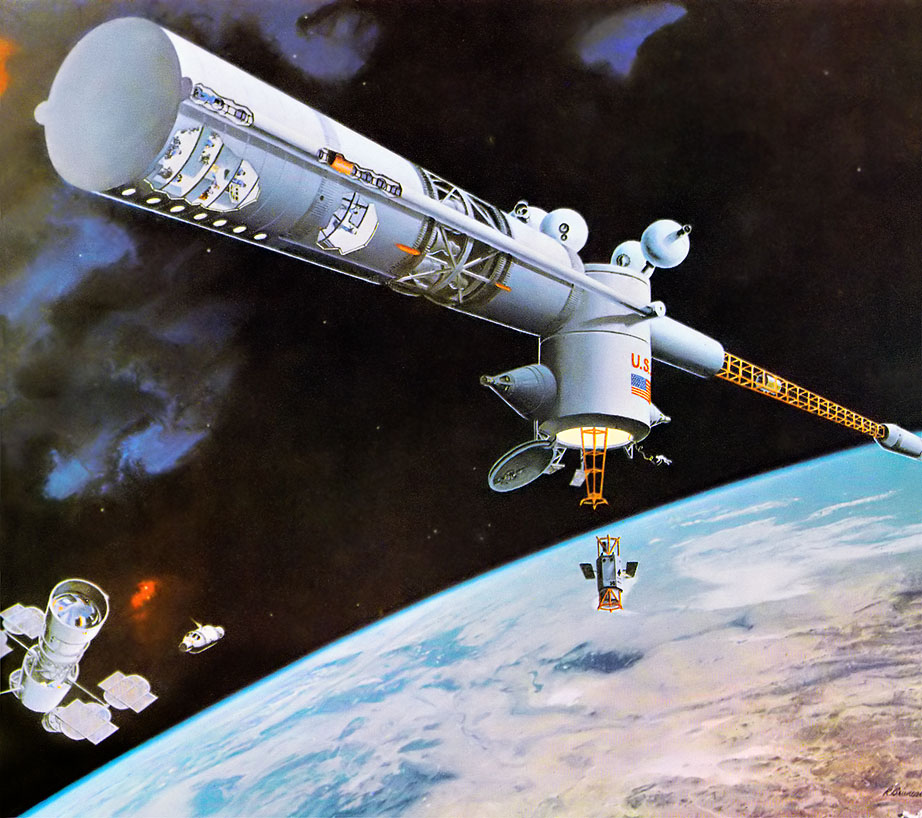This is a detailed and vibrant cartoon drawing of a space scene featuring a large, industrial-looking space station prominently in the center. The backdrop consists of the Earth, which is vibrant and well-lit, showcasing distinct land and water masses. The dark, cosmic sky behind Earth transitions into purple and black hues, interspersed with stars, a red blob, and a blue aurora-like feature in the upper left-hand corner.

The central space station is grayish-white with elements that make it appear industrial, including a noticeable yellow metallic ladder or bridge section and orange fencing. The structure is composed of several cylindrical components, suggesting a complex and modular design. One part of the space station is shown with a round opening, and something appears to be floating out from this section. The illustration gives a glimpse of the interior through a circular tube-like structure with a wall partially removed, revealing the inner workings.

In the bottom left corner, there is another significant object that could be a space station or satellite. This object is also white, somewhat cylindrical, and appears to have a large telescope or sonar detection equipment attached to it, adding to the scientific and exploratory theme of the image. The meticulous details, such as the open cylindrical compartments and floating elements, offer a dynamic and captivating depiction of space exploration.